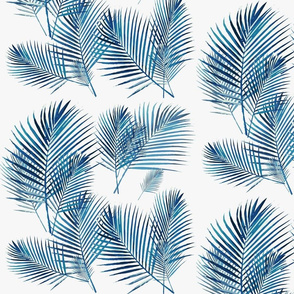The square image showcases a detailed depiction of a plant pattern on an off-white background, creating a delicate and artistic composition. The primary elements appear to be large frond-like leaves, arranged diagonally from a central stalk, forming a 90-degree angle when paired. These leaves are not the typical green but instead vary in hues of dusty blue, medium blue, and dark blue. The image has a sun print or digital stamp effect, giving the impression of fine etching or photographic imprinting. There are approximately 15 leaves in total, set up in three inconsistent rows. Each row features leaves of differing sizes, from small to medium to large, without a consistent arrangement. This creates an intricate visual pattern that is both organic and meticulously designed.